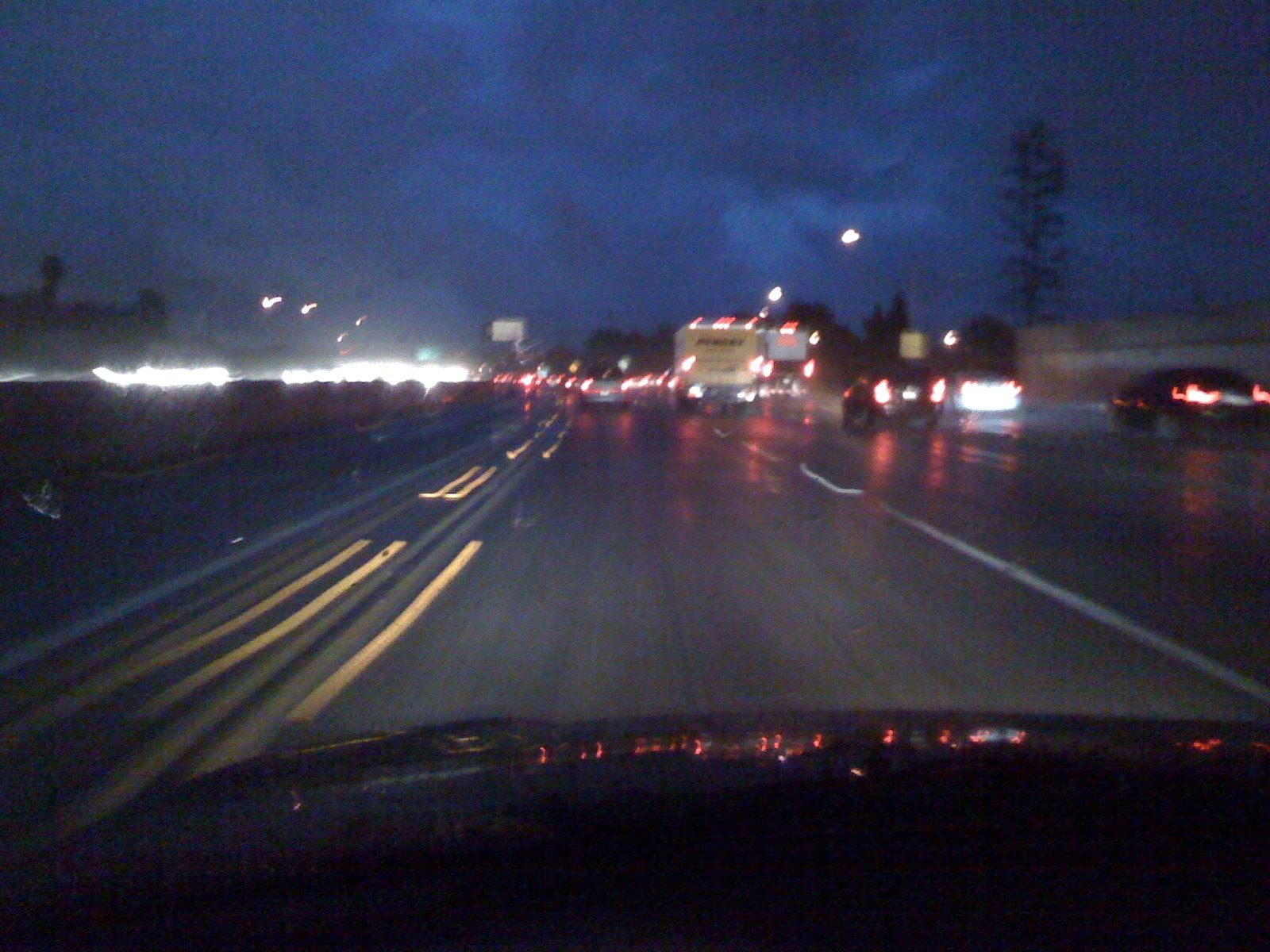This nighttime highway scene captures the blur of movement from a vehicle in motion. The image, slightly blurry due to the car's speed, showcases a bustling road full of vehicles. On the opposite side of the highway, a line of bright headlights glows intensely, contrasting with the darkening sky that transitions from deep blue to black, partially veiled by clouds. Streetlights appear as streaks of light, enhancing the sense of speed. Ahead, numerous cars with glowing red brake lights indicate heavy traffic and cautious braking. The road itself has a reflective sheen, hinting at recent rainfall, which adds a shimmering texture to the scene despite the absence of visible windshield wipers.